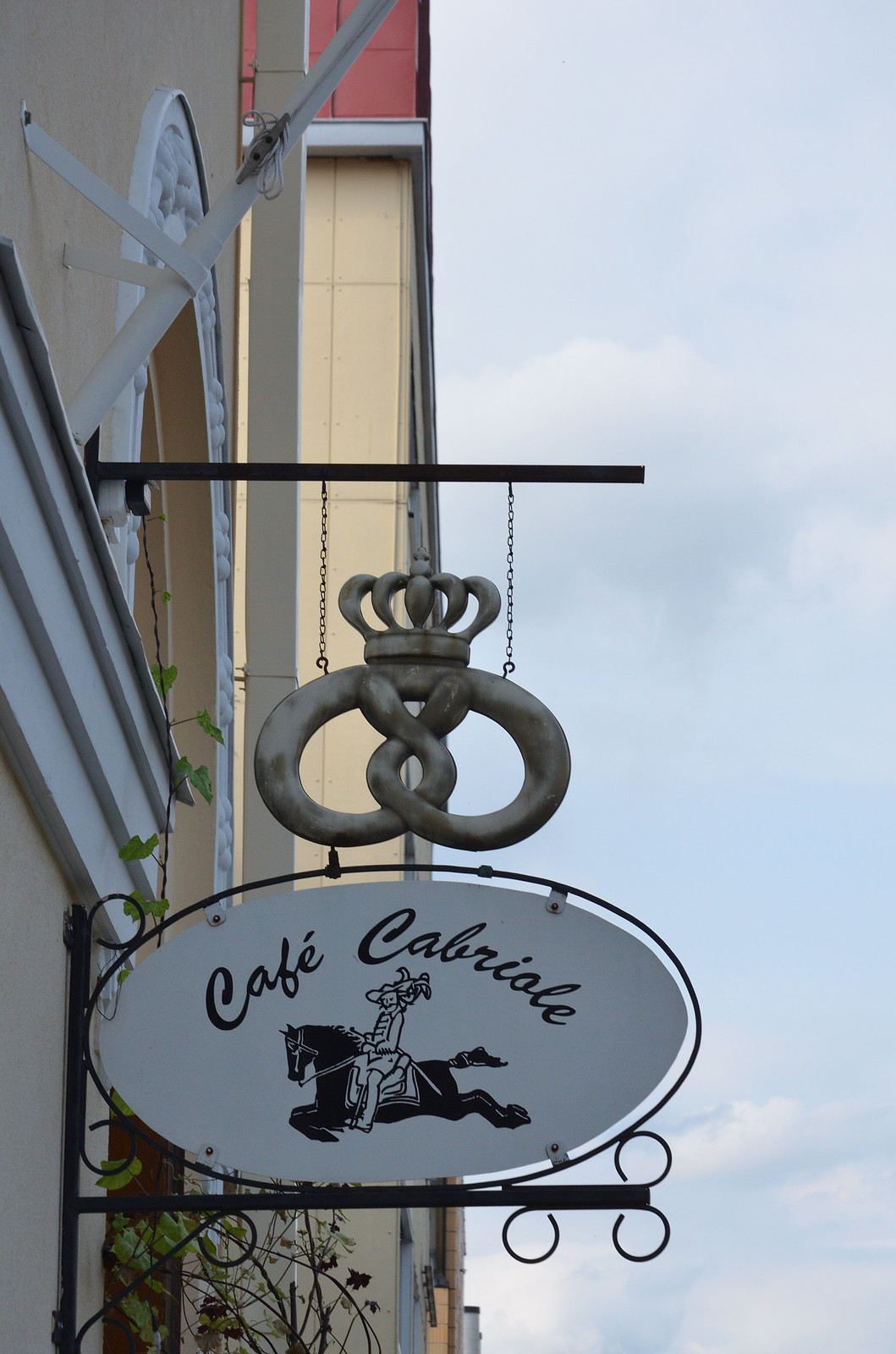The image captures an outdoor scene featuring a detailed metal shop sign suspended from a building facade. The photograph is taken from a low angle, giving the perspective of someone standing on the sidewalk beneath the sign. The sign is comprised of two main sections: the upper part features an intricate metal Celtic knot design, resembling a large, silver-gray pretzel crowned with a decorative element, all suspended by chains from a black horizontal bar jutting out from the building. Below this, another horizontal bar, adorned with curl designs, supports a white oval sign depicting a man riding a galloping black horse, with its tail flared and legs extended mid-jump, facing left. Above this oval illustration, the text "Cafe Cabriolet" is elegantly scripted in black, curved along the top edge of the oval. The background on the left side consists of a tan-colored building facade with a white arch decoration above, while the right side of the image is dominated by a blue sky with wisps of thin, white clouds and some grayer patches at the top. Another building, taller and with yellowish walls, is visible behind the first building, with a small silver-gray bar protruding from its top. The composition overall captures a blend of architectural details and the striking design of the hanging sign against a picturesque sky.